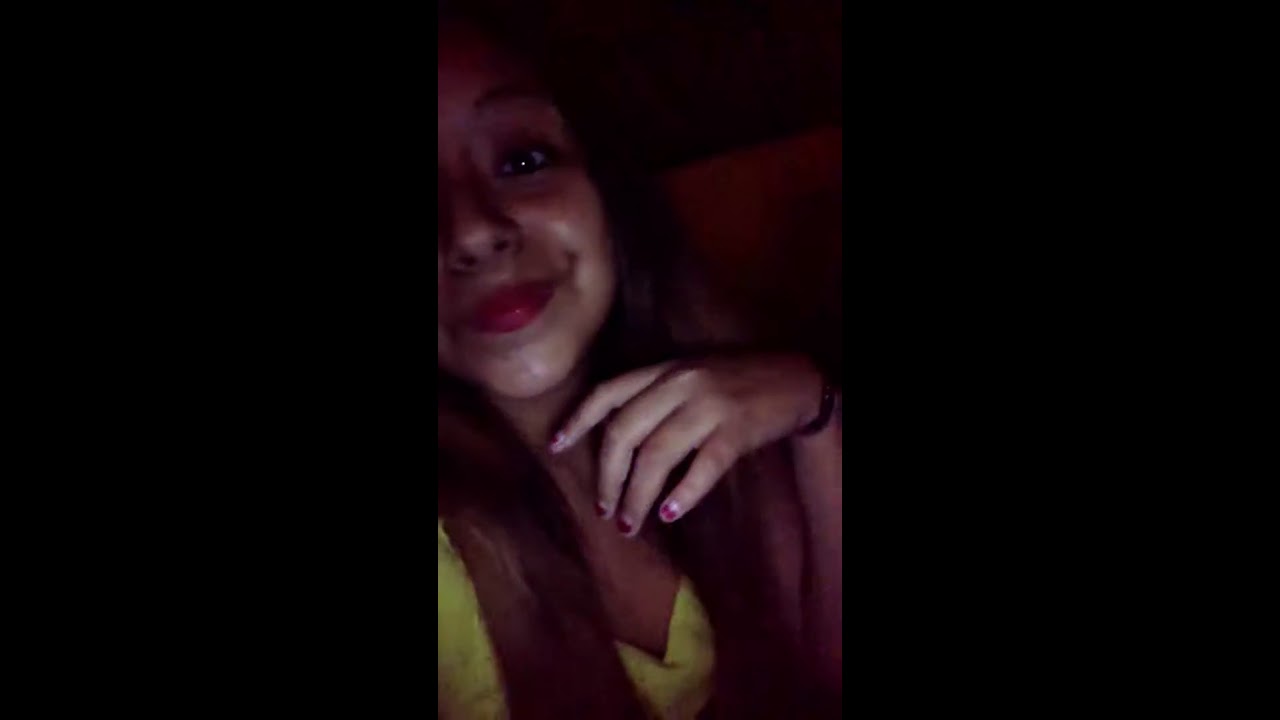This rectangular, horizontally-oriented photograph features a young adult woman, possibly of Indian or Hispanic descent, set against a completely dark background with the left and right thirds of the image filled by blackness. She is positioned off-center, with the top left of the frame cutting off half of her face, obscuring her right eye. Her visible left eye is wide open, and she has a closed-mouth smile highlighting her full, vibrant red lips. Her long, straight brown hair cascades down her shoulders. The woman is wearing a bright, neon-yellow v-neck top. One of her arms is raised, with her left hand just beneath her chin. Her fingernails are partially painted red with visible chipping, and she is adorned with a black bracelet or possibly a watch on her wrist. The image, poorly lit and seemingly taken indoors at night, depicts her in a warmly expressive, though somewhat mysterious and shadowy, pose.